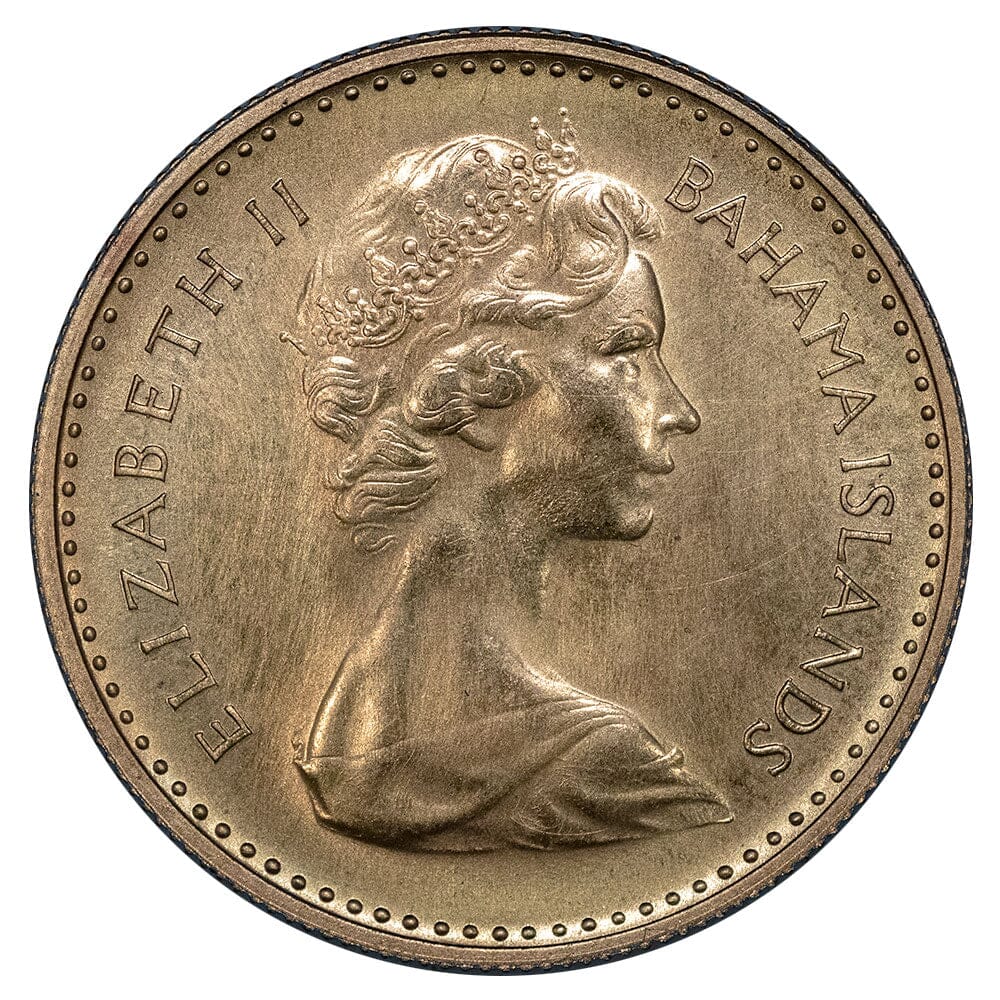This close-up image showcases a coin from the Bahama Islands, primarily gold or copper in color, though it's slightly dingy which makes the exact material difficult to ascertain. The coin rests on its side, presenting an enlarged view of its intricate details. Encircling the outer edge, a thin copper rim is bordered by a series of fine, raised dots. At the heart of the design is a side profile portrait of Queen Elizabeth II, depicted from the shoulders up. She faces to the right, adorned with a crown that diagonally spans from the top right of her head down to the bottom left. Her features include a pointy nose, long neck, and short hair etched carefully into the coin. Draped over her shoulders is a small shawl. Behind her head, following the curve of the coin, the inscription "Elizabeth II" is engraved on the left side, while "Bahama Islands" appears above her forehead on the right. The coin, showing signs of wear with minor scratches, lacks a polished finish, resting against a stark white background.